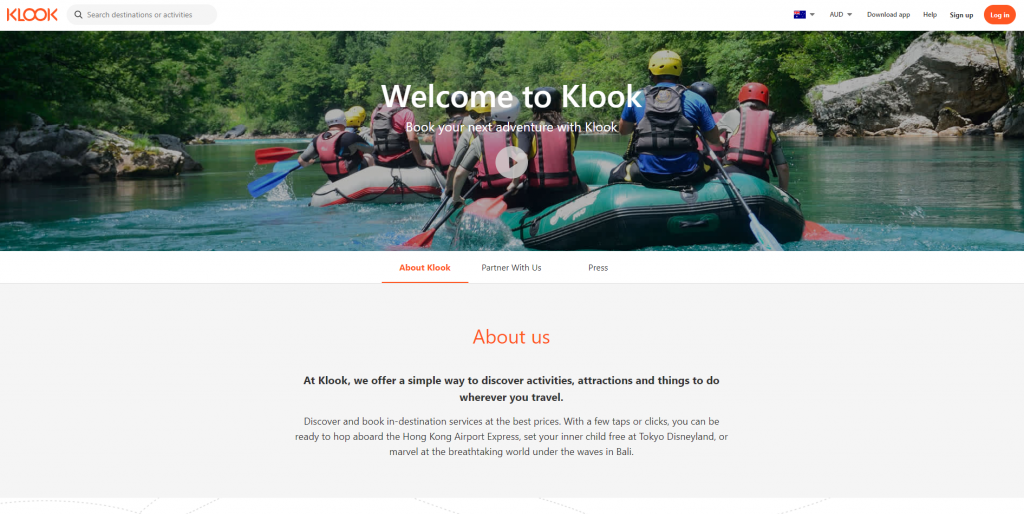The top-left corner of the image features the Klook logo in bold orange letters. To its right, there is a search bar. Positioned on the top-right are options for selecting the language and currency (with AUD displayed), alongside links for downloading the app, getting help, signing up, and logging in. The "Login" option stands out in orange.

Centrally, the text "Welcome to Klook. Book your next adventure with Klook" is prominently displayed. Below this, there are vibrant images of people paddling boats on a lake, donned in red life jackets. The boats are a mix of green and black, and grey and red. Participants are equipped with helmets in various colors, including white, red, black, and yellow. 

The background scenery showcases lush green trees lining the front of the lake. Beneath this visual, the text sections include "About Klook," "Partner with us," and "Press," with "Airport Look" highlighted in orange while the others are in black.

Towards the bottom, a detailed description reads:
"At Klook, we offer a simple way to discover activities, attractions, and things to do wherever you travel. Discover and book in-destination services at the best prices. With just a few taps or clicks, you can be ready to hop aboard the Hong Kong Airport Express, access your inner child at Tokyo Disneyland, or marvel at the breathtaking world under the waves in Bali."

The description text is mainly in black, except for "About us," which is highlighted in orange. The entire image background is white, creating a clean and visually appealing layout.